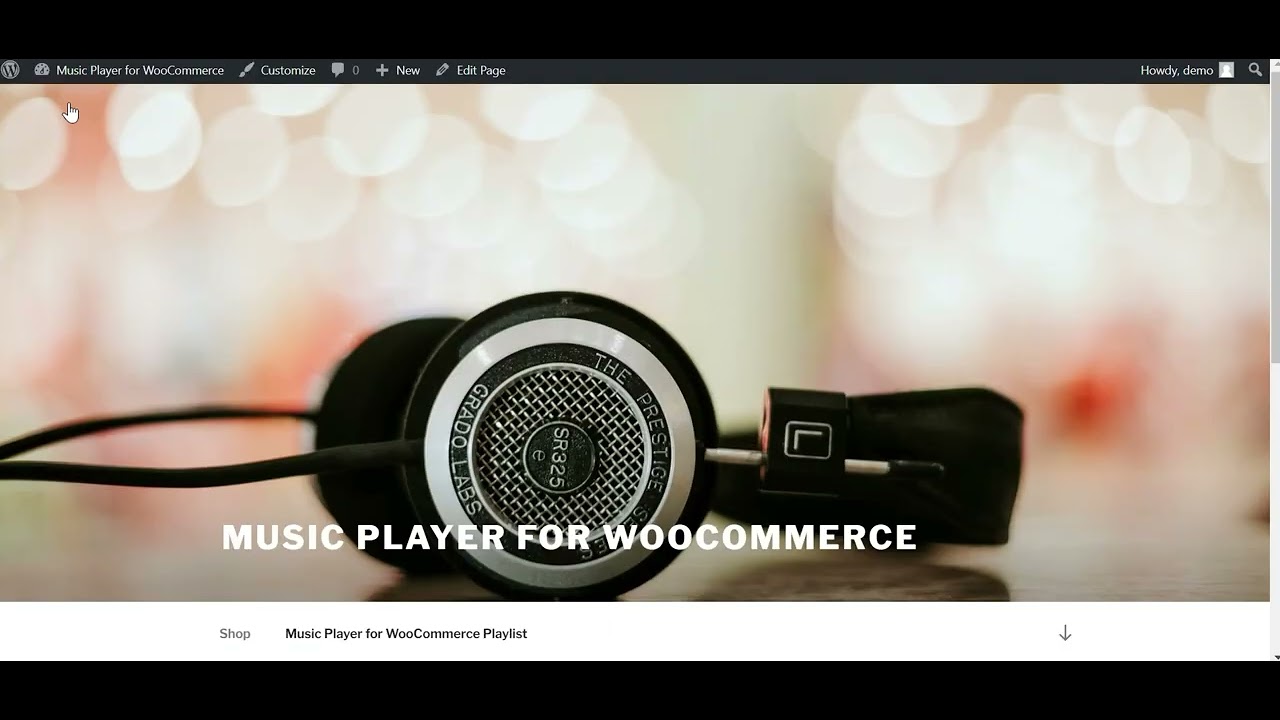The image showcases a detailed webpage with a set of over-the-ear headphones prominently displayed in the foreground. The headphones are black with silver or white accents and are labeled "The Prestige Grotto Lab." The specific pair shown is positioned on a table, revealing the left side with an "L" symbol denoting the left ear speaker.

In the background, the webpage features a black and white theme with black borders at the top and bottom. The top section includes a white border that displays navigational text: "Shop" and "Music Player for WooCommerce." Central to the page's content area, there is text reading "Music Player for WooCommerce" with a "Shop" button below it. To the right of the button, there's a downward-pointing arrow, indicating additional options or a menu. 

Additional elements on the page include a blurred background with indistinguishable lights, creating a focused view on the headphones. At the top of the page, there are options for customization and editing, indicated by the text "Customize," a chat icon, a plus icon, and an edit page icon. The upper right corner features a welcome message, "Howdy Demo," accompanied by a user avatar placeholder.